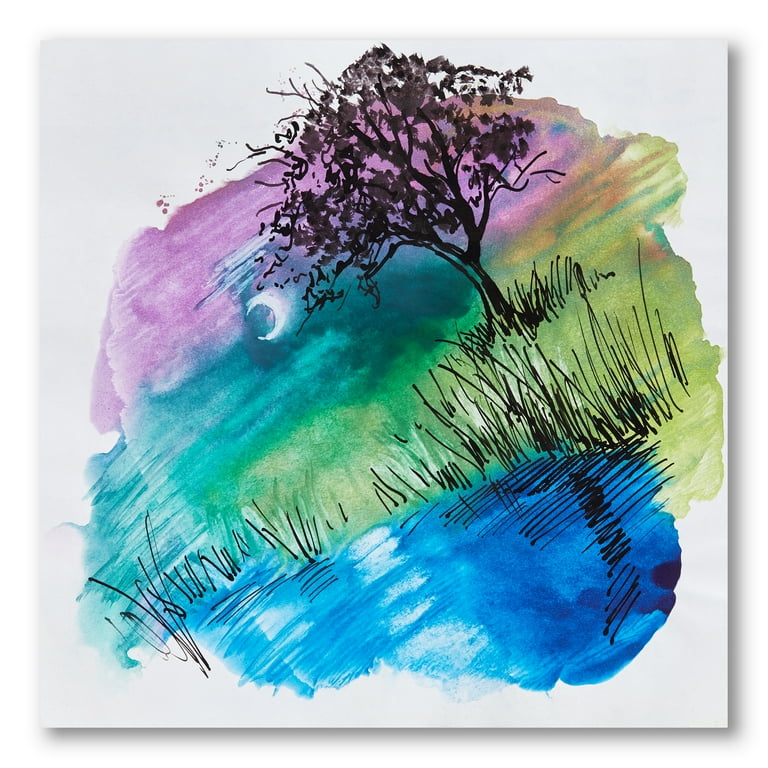This image features a square white canvas with a simple mixed-media painting, combining both watercolor and pen. The scene on the canvas shows an angular tree, positioned diagonally from the lower left corner, ascending upwards to the middle of the right side. The tree, rendered in bold black, is partially leafless yet still holds numerous mauve-colored watercolor leaves. Below the tree, there is a blue streak indicative of a water's edge, with black pen marks representing tall grass or reeds rising from the water. The sky above displays a vibrant blend of watercolors, transitioning from purplish-pink at the top to teal on the left, and orange and yellow hues on the right, concluding in deep green shades closer to the tree. A rich blue color at the bottom complements the scene. Adding to this somewhat abstract representation, a white moon is visible between the purple and teal areas, enhancing the overall impressionistic lakeside or pond-side atmosphere. The entire artwork is mounted on a white wall, with a subtle drop shadow framing the canvas.